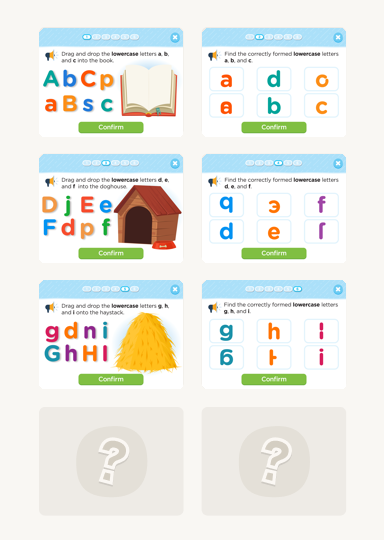This image, captured from a digital screen, appears to be an educational tool intended for preschoolers to practice their alphabet skills. The interface resembles a long, narrow rectangle, similar in shape and size to a smartphone screen. The screen is divided into eight sections for interactive cards, but the bottom two spaces are blank and gray, each featuring a circle with a question mark inside — indicating they may be for additional content or placeholders.

The first six sections display interactive cards aimed at teaching lowercase letters A, B, and C. The top card instructs the child to drag and drop lowercase letters A, B, and C into a virtual book. On this card, the following letters are available to choose from: uppercase A, lowercase B, uppercase C, lowercase P, lowercase A, uppercase B, lowercase S, and lowercase C. A book icon on the right side of the screen shows an open page where the selected letters should be dragged and dropped. Below this book icon, there is a green rectangular button labeled "Confirm" for the child to submit their answers.

Each subsequent card follows a similar format but with different instructions, such as finding correctly formed lowercase letters A, B, and C. Each card features a similar setup where children can interact with letters and a confirm button to verify their choices, providing a structured and engaging learning path for mastering basic alphabet skills.